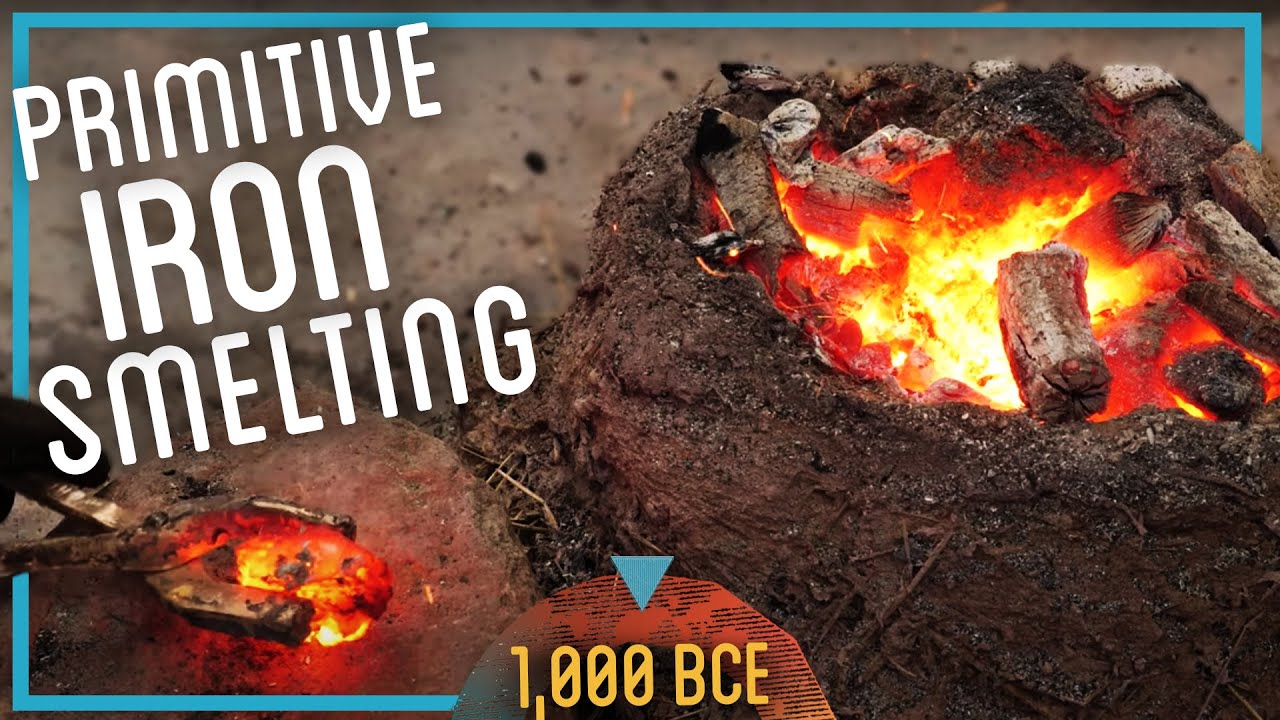The image, which is wider than it is tall, depicts a scene labeled "Primitive Iron Smelting" in white text at the top left. Framed with a blue border, the photograph features a dirt mound serving as a rudimentary furnace filled with charred wood and glowing red and yellow embers, used to generate the high heat necessary for smelting iron. On the left side of the image, a black-gloved hand is holding large iron smelting pliers, gripping a piece of iron that is glowing red hot. At the bottom center of the image, gold text reads "1000 BCE," indicating the historical period being illustrated. The overall composition vividly conveys the ancient techniques of iron smelting, highlighting the tools and conditions used in the process.